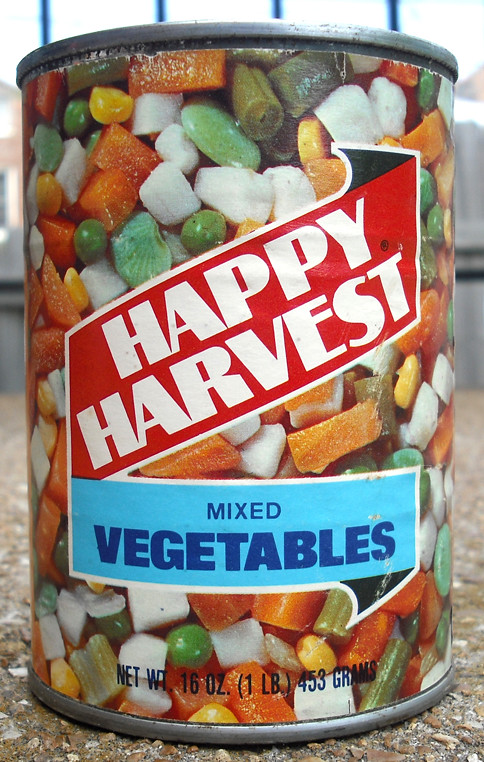The image features a vintage, slightly rusted can resting on a piece of granite. The granite itself has a complex pattern composed of miniature stones in various shades of brown and gray, with a striking white top surface. The old can bears a colorful label with illustrations of assorted vegetables, including orange, white, green vegetables, and yellow corn, creating a vibrant mix. Encircling the top of the can is a tarnished silver rim. The label also includes detailed text: "Net Weight: 60 ounces (1 pound, 453 grams)" is prominently displayed. At the top of the can, a red banner with white text reads "Happy Harvest." Near the bottom of the can, a light blue rectangle contains the words "Mixed Vegetables," providing additional context to the can's contents.